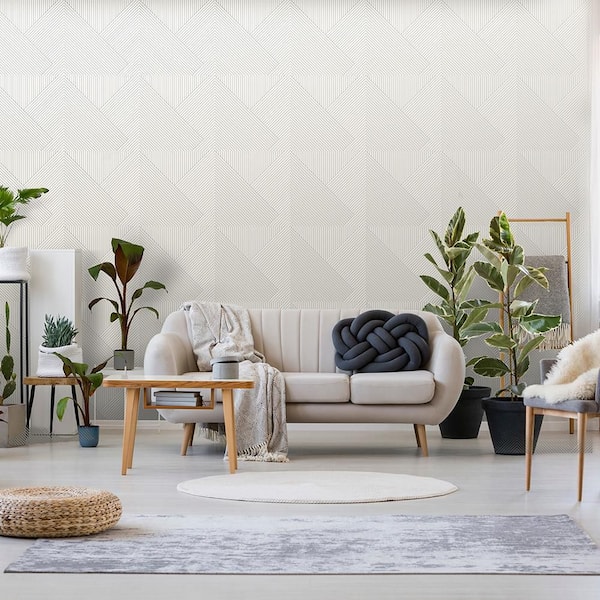This color photograph captures a modern, cozy, and sophisticated living room with a serene color palette centered around shades of white, gray, and beige. The main focus is an ivory-colored, plush sofa with four wooden peg legs. Adorning the sofa are a contrasting dark pillow, designed to look like a knotted piece of rope, and a draped white throw blanket. 

Adjacent to the sofa, a low-to-the-ground, beige, straw-like cushion rests. The room's flooring appears to be polished concrete, partially covered by a textured, gray area rug with cream accents. A smaller, white circle pattern adds detail to the rug.

In front of the sofa stands a modern, wooden coffee table with thin legs and a white top bordered by light wood. It holds a few decorative items, emphasizing the room's contemporary aesthetic. To the right side of the sofa, near the horizontal photograph's edge, leafy plants in black pots add a touch of greenery and freshness, complemented by another low potted plant closer to the left.

A white chair with wooden legs and a fur-covered seat sits comfortably within the space. Completing the backdrop, the wall behind the sofa has a subtle pattern of white-on-white squares creating a chic yet understated visual interest. A sleek, tall mirror with a thin light wood frame also stands on the right side of the photo. 

Overall, this room's design blends minimalistic modern elements with touches of warmth and texture, creating a lived-in yet stylish environment.